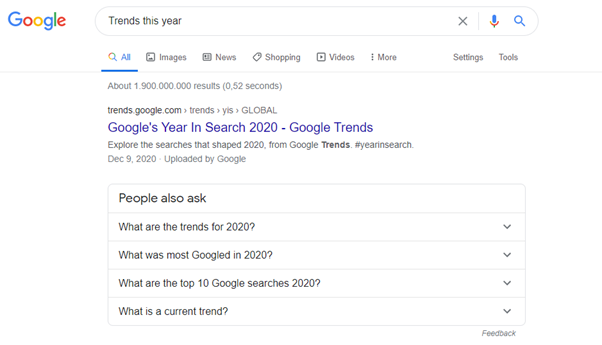This screenshot captures a Google search results page with a predominantly white background. In the upper left corner, the iconic Google logo is prominently displayed, featuring the word "Google" in its signature multicolored primary hues. Adjacent to the logo is the search bar where the query "trends this year" has been typed. At the end of the search field, on the right side, are a blue magnifying glass icon, a microphone icon, and an 'X' for clearing the search input.

Directly beneath the search bar, a menu with various options is visible in gray font, including "All," "Images," "News," "Shopping," "Videos," "More," "Settings," and "Tools." A thin gray line separates this menu from the search results below. The search engine indicates that there are about 1,900,000 results for the query, retrieved in 0.52 seconds.

The first search result is from "trends.google.com" and is broken down as follows:

- In smaller gray text: "trends.google.com › YFS › global"
- In larger blue font: "Google's Year in Search 2020 - Google Trends"
- In gray text below the title: "Explore the searches that shaped 2020 from Google Trends. #YearInSearch December 9th, 2020, updated by Google."

Further down, there is a section titled "People also ask," featuring expandable questions like "What are the trends for 2020?" and "What was the most Googled in 2020?"